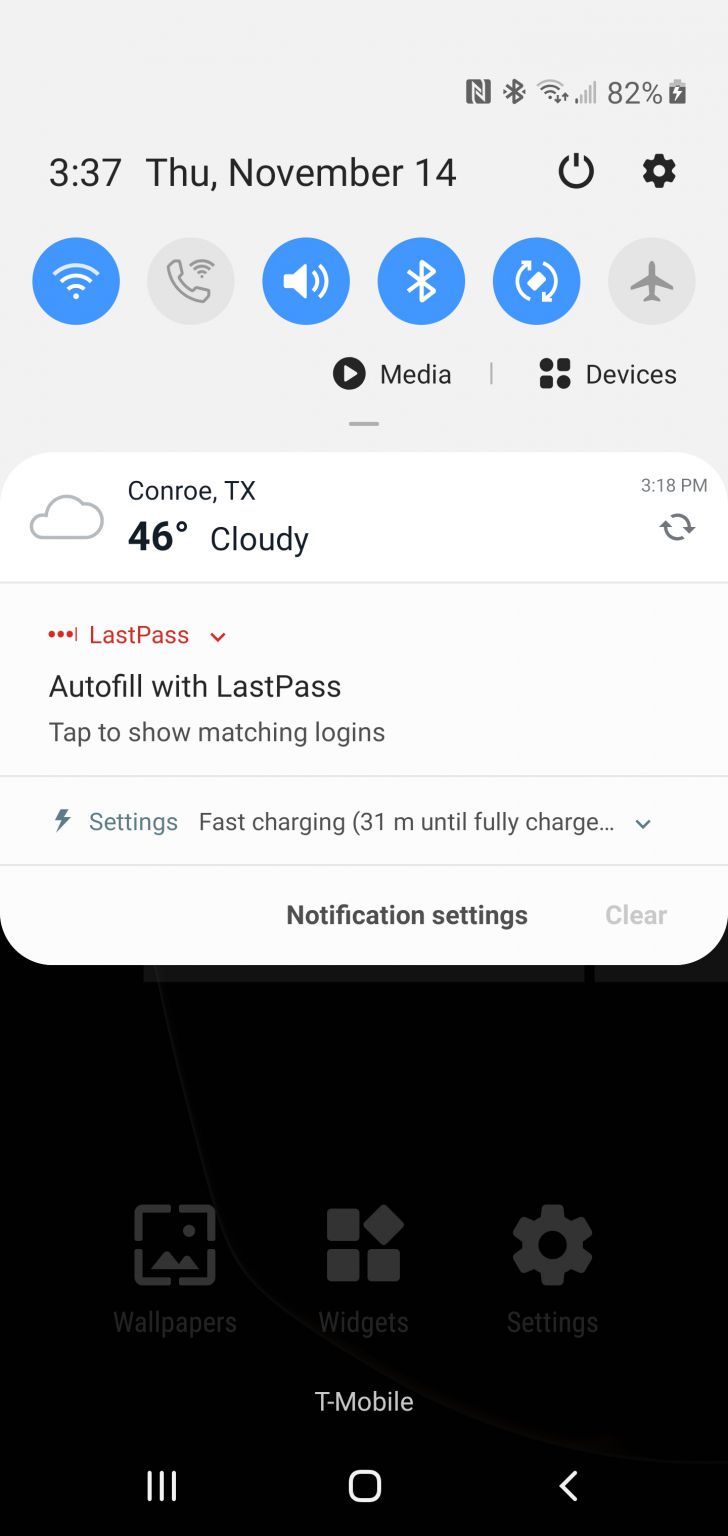In this image from a T-Mobile phone, the status bar at the top displays an 82% battery level, three out of four bars for internet connectivity, and one bar for phone signal. The time shown is 3:37 PM on Thursday, November 14th. Below this status bar, there are quick access options for internet, making a call, adjusting volume, Bluetooth, and airplane mode. Four of these options are highlighted in blue, while the phone call and airplane icons are grayed out. 

Further down, the screen features the labels 'Media' and 'Devices.' The weather update indicates it's 46°F and cloudy in Conroe, Texas, last updated at 3:18 PM. The 'LastPass' section in red offers autofill for matching logins with a prompt to tap. Below, there's a notification for fast charging, indicating 31 minutes remaining until fully charged. Additional options for notification settings and a clear button are visible.

At the bottom of the screen, there's a black square with 'T-Mobile' centered. Three icons beneath this square provide shortcuts to Settings, Widgets, and Wallpaper.